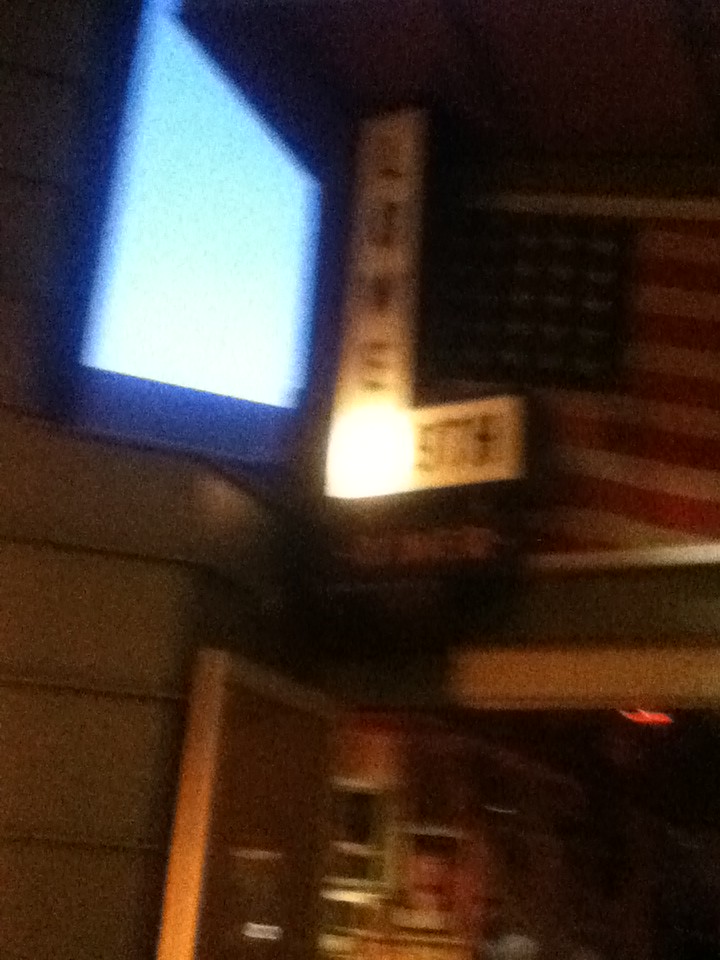The image portrays a somewhat blurry interior of an establishment, possibly a restaurant, with a focus on several distinct elements. On the left side, there's a dark wall adorned with vertical wood slats, topped with a mounted flat-screen TV displaying a blank blue light screen and surrounded by a dark blue trim. Adjacent to the TV is a prominent L-shaped sign featuring Asian-style writing; it extends from the top of the screen downwards and includes a mix of dark lettering on a white background. Below this sign, there's an illuminated area obscured by bright light, making it difficult to discern specific details. At the top center of the image is a partially visible American flag, showing the blue field and a portion of the red and white stripes. Underneath the flag, a doorway frames a transition into another room, dimly lit compared to the bright area in the foreground. The overall impression is that of a complex scene with multiple layers of visual interest, despite the image's blurry quality.